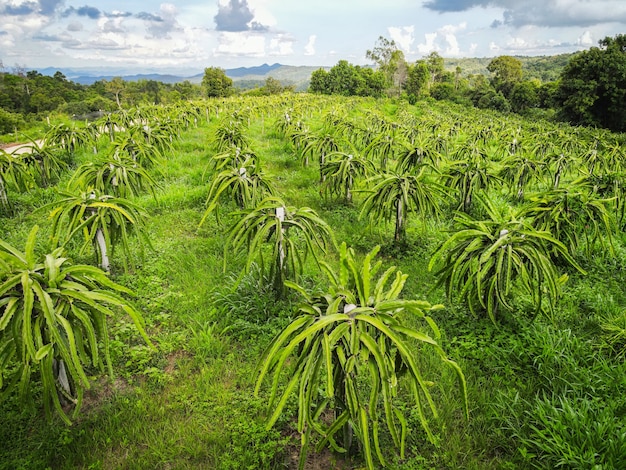The image captures an expansive, lush field that appears to be a type of farm specializing in dragon fruit cultivation. The ground is carpeted with vibrant yellowish-green vegetation, and the scene is bathed in a mix of sunny light and overcast skies with white and gray clouds. In the foreground and stretching into the distance, there are at least ten neatly aligned rows of dragon fruit plants. Each plant is supported by a wooden post, with long, snake-like leaves or stems draping over the top, resembling the fronds of a palm tree but with a distinctive yellowish-green hue.

The plants are arranged in a consistent triangular pattern with pointed tips along the leaves' edges, typical of cactus species. The rows are interspersed with green grass, enhancing the lushness of the field. Surrounding the cultivated area, large green trees form a natural border, while distant mountains add a picturesque backdrop to the setting.

Despite the abundance of vibrant flora, there are no dragon fruits visible on the plants, nor are there any people or structures like barns in sight. A road runs down a hill on the top left corner of the image, marking the periphery of this serene agricultural landscape.